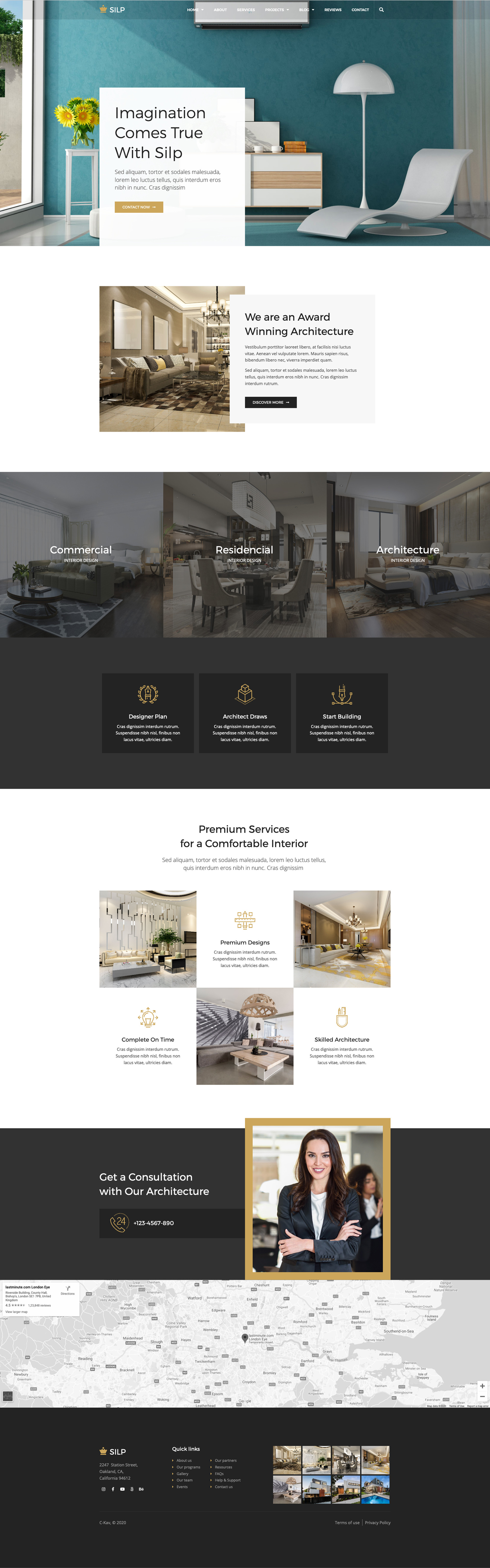**Website Screenshot Description:**

The screenshot showcases the homepage of SILP, a website dedicated to architecture and interior design services. In the top left corner, the SILP logo is prominently displayed, featuring a gold bathtub silhouette. Overlaying the top of the page is a transparent navigation bar that provides links to various sections: Home, About, Services, Projects, Blog, Reviews, and Contact. It also includes a search bar.

Dominating the topmost part of the page is a visually striking image of a wavy, modern-style lounge chair set against a teal wall. Complementing this scene is an array of white furniture. Superimposed on this image is a white text box that reads, "Imagination comes true with SILP." Below this primary message, there is additional text in a different language, alongside a "Contact Now" button.

Immediately beneath this section, there is another highlighted box proclaiming, "We are an award-winning architecture." A black link within this box invites users to "Discover More."

The following section systematically categorizes SILP's offerings into three main areas: Commercial Interior Design, Residential Interior Design, and Architectural Interior Design. Further options branching out from these categories include "Designer Plan," "Architect Draws," and "Start Building."

Moving down, the next segment emphasizes the premium nature of SILP’s services with phrases such as "Premium services for a comfortable interior," "Complete on time," "Premium design," and "Skilled architecture."

At the bottom of the page, there is a contact phone number and an image of a woman in a suit standing confidently with her arms crossed. Adjacent to her image is an embedded map, ostensibly showing the company's location. Finally, the footer of the webpage offers quick links or a site map for user convenience.

This detailed depiction effectively encapsulates the essence of the SILP website, ensuring that users understand its structure, offerings, and visual appeal.